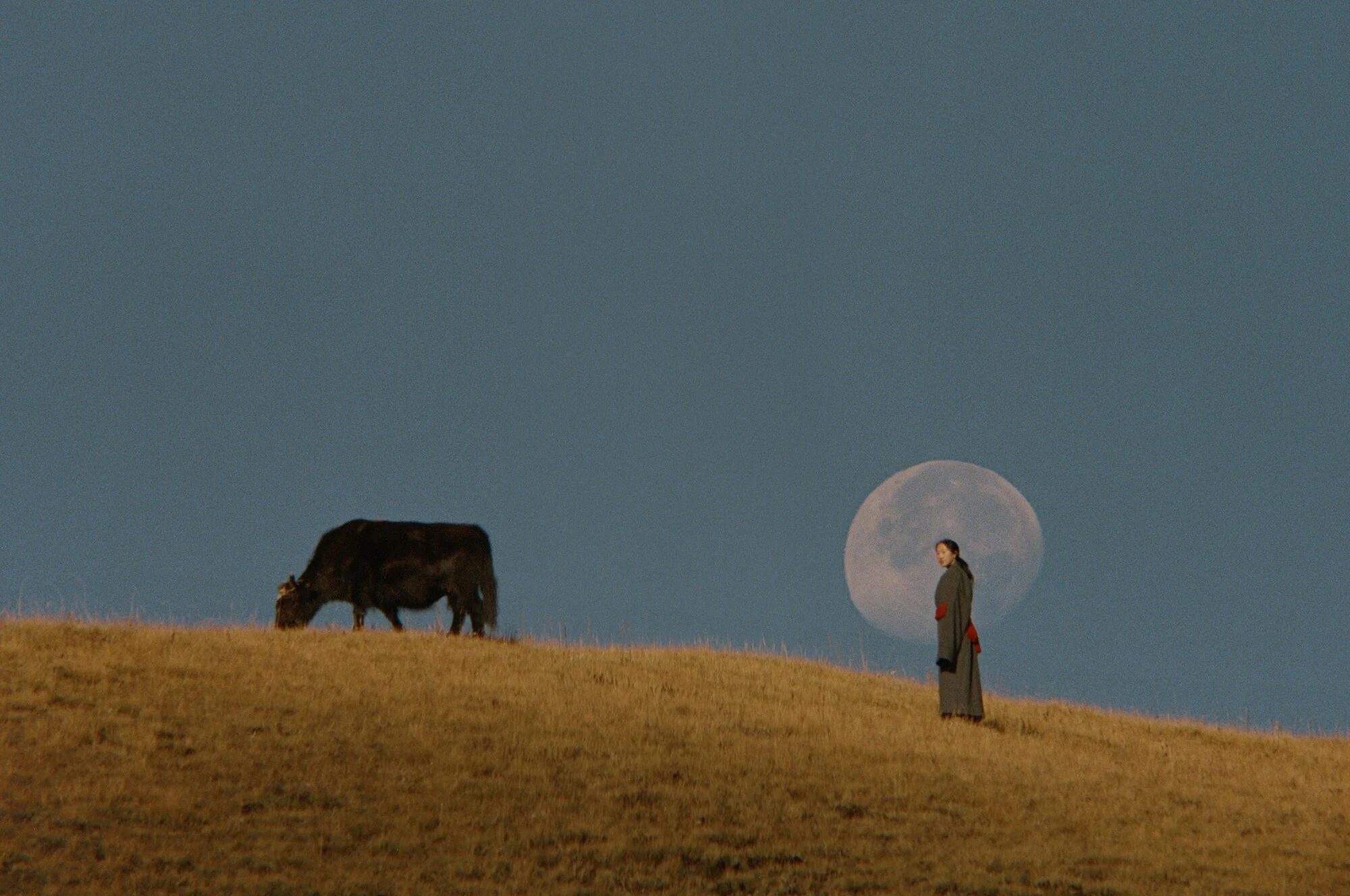In this evocative image, a woman stands solemnly on a barren hilltop under a dark gray sky. She is dressed in a long, dark gray robe, cinched at the waist with a vibrant red sash that trails down her back, possibly invoking the aesthetic of a traditional uniform or garment. Just ahead of her, several feet up the hill, is a fully brown cow, contrasting with the more commonly recognized black and white variety. The cow appears to be foraging on the sparse, dark brown grass that sparsely covers the hill. The woman is centered perfectly in front of the rising moon, creating an almost ethereal halo effect around her, suggesting a carefully composed scene that could easily be a still from a movie. The landscape appears desolate, adding to the surreal, almost mystical atmosphere of the photograph.